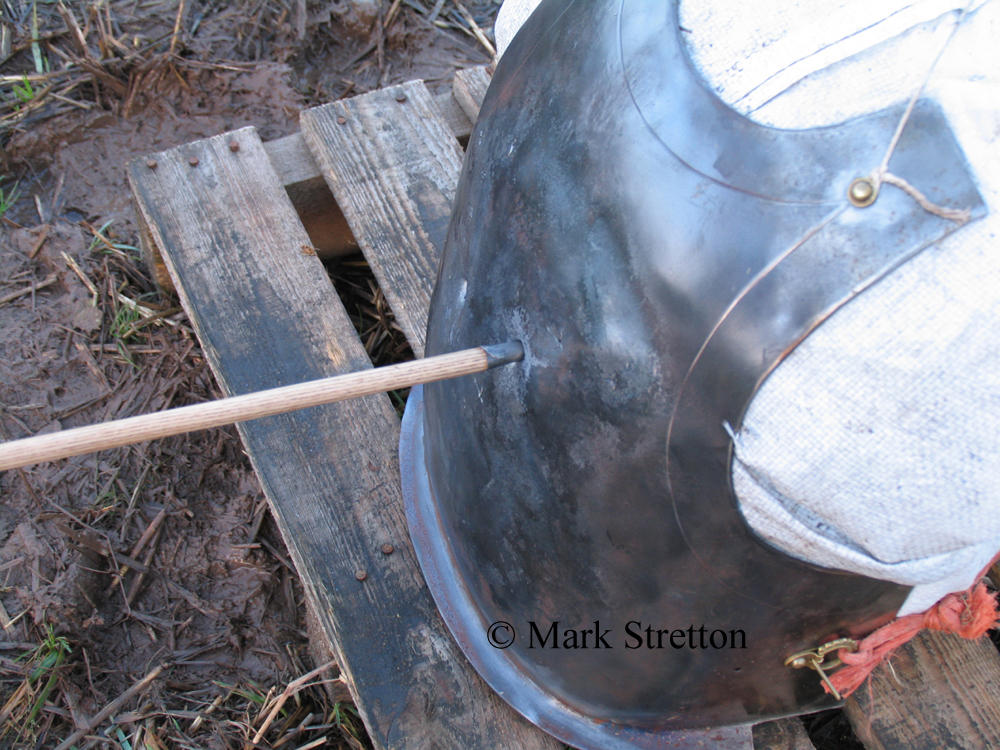The photograph, taken by professional photographer Mark Stretton, captures an outdoor scene featuring a chest armor piece, possibly a breastplate, used by soldiers in battle. The image showcases a wooden pallet, which is worn and old, set amidst a muddy terrain with sparse grass and plants. Centrally positioned on the pallet is the breastplate, slightly to the right in the frame. The armor, rounded at the shoulders and extending from below where the stomach would be to the upper chest, is depicted as being pierced by an arrow. The arrow, with its metallic tip, is embedded almost directly in the center of the armor, suggesting a target practice scenario or testing of the chest plate’s durability. The lower part of the image contains a copyright attribution to Mark Stretton. The color palette includes shades of brown, beige, black, white, gray, orange, and light blue, indicative of the natural outdoor lighting and the earthy setting of this rustic scene.